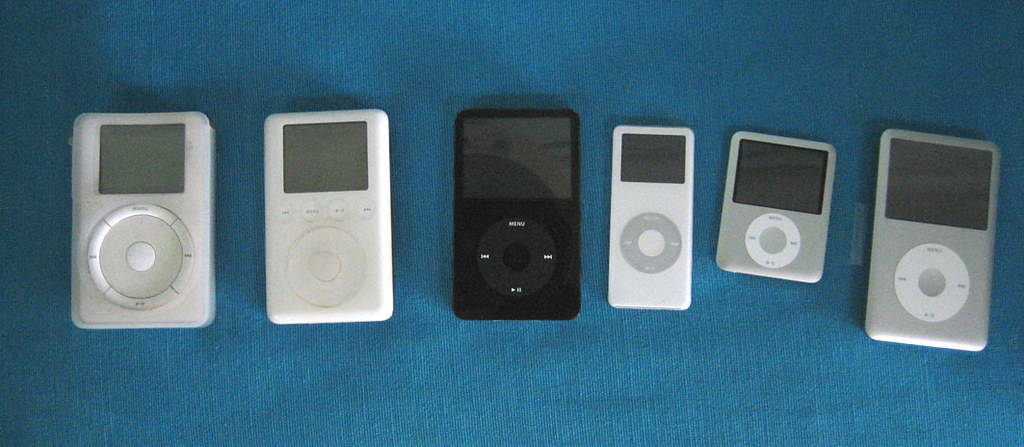In this photograph, six iPods of varying sizes and shapes are neatly arranged from left to right on a medium blue upholstery background that resembles denim. The first iPod on the far left is a thick, white model featuring a large dial with raised buttons including forward and reverse controls, and a gray screen. Next to it is a slightly smaller white iPod with rounded edges that features a flat touch ring and four round buttons situated above a square gray screen. The third iPod in line is a black model with a touch ring labeled "Menu" and includes skip buttons and a play/pause button at the bottom of the ring. 

The fourth iPod is a very slim, white device with a gray control ring at the center. To its right, there is a shorter, wider silver iPod with a central white ring. The last iPod on the far right is a large silver model, characterized by rounded corners, a white control ring, and a large gray screen. The blue upholstery backdrop provides a cohesive visual element that highlights the differences in design and size of each iPod.